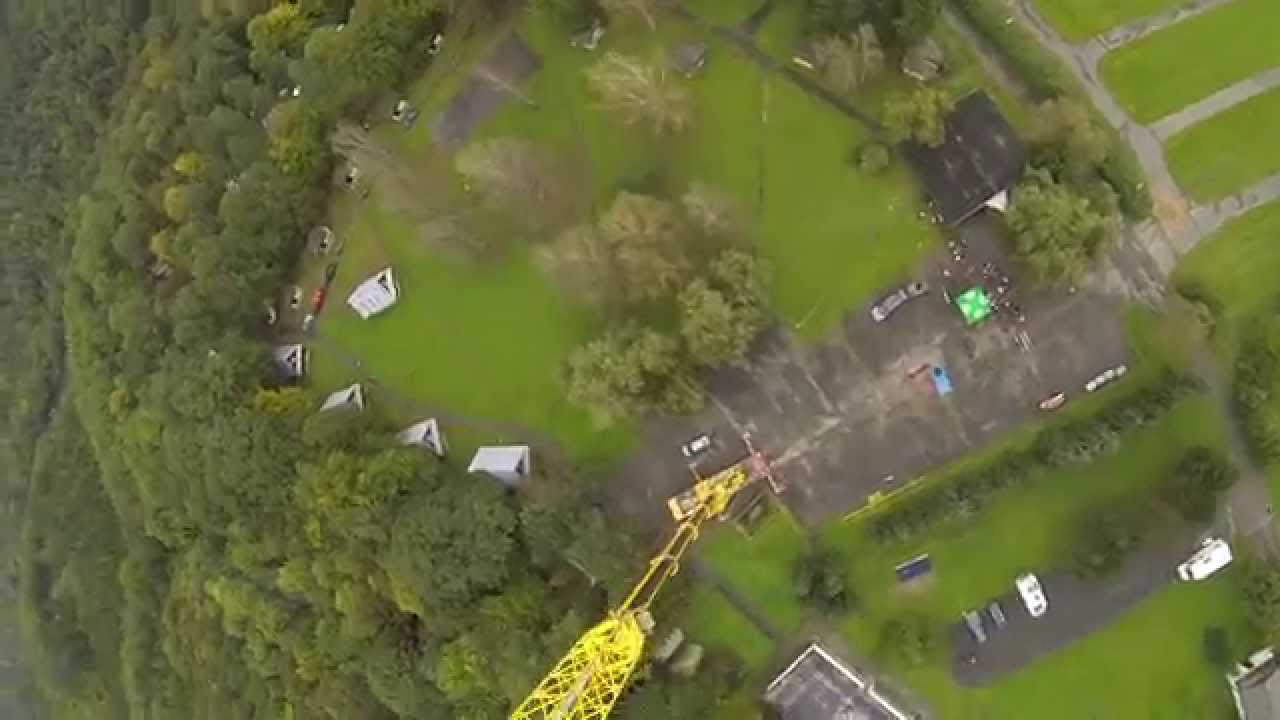This aerial photograph, likely captured from a high vantage point such as a drone, aircraft, or perhaps the top of a yellow metal tower visible at the bottom of the image, reveals a detailed and vibrant scene below. Dominating the left side and central portion of the photo is a dense half-circle of green trees surrounding a clearing with lush grass. Nestled along the periphery of this clearing are five distinctive white triangular structures that resemble tents. In the middle of this area, you can spot a smattering of trees, approximately seven or eight.

The yellow metal tower, which extends from its base in a black paved parking lot and rises out of the photograph, stands prominently at the bottom. Adjacent to this tower, there are several vehicles, including a blue car, a white car, a camper, and a few others scattered around the parking space. At the bottom right, a separate driveway contains four more vehicles.

On the right-hand side of the image, a series of dirt access roads weave through green fields and past a larger structure, possibly a house or another significant building, located at the top-right corner of the photo. This building is connected by a pathway emanating from its entrance. Additionally, a canopy tent marked with a green cross is noticeable, along with a gathering of people nearby. The dominant colors of the scene are a vibrant mix of green, white, gray-black, and the striking yellow of the tower, providing a rich visual contrast in the landscape.